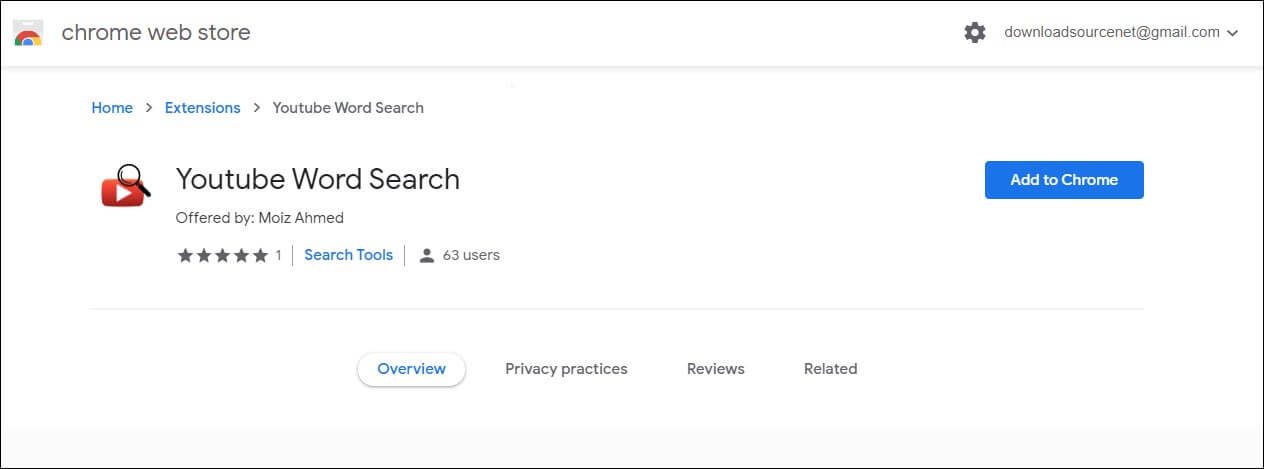The image depicts the Chrome Web Store interface. At the top left corner, the Chrome Web Store logo is visible with the text "Chrome Web Store" displayed in gray. Adjacent to the text, there is a small Chrome symbol. On the top right, there is a gear icon representing settings, followed by an email address "download-source-net@gmail.com" written in gray, accompanied by a downward-facing arrow.

Below the top bar, navigation links are highlighted in blue, starting with "Home," followed by an arrow, then "Extensions," and another arrow leading to "YouTube Word Search" in gray. Beneath this, in larger black text, the title "YouTube Word Search" is prominently displayed. To the left of this title, there is a small icon featuring the red YouTube play button with a white triangle in the center, overlaid by a black magnifying glass symbol.

On the right side, the plugin is noted to be "Offered by Moiz Ahmed." Below this, five gray stars are displayed with a "1" next to them, indicating the rating. In blue text, the category is identified as "Search Tools." To its right, a small gray icon of a person is displayed with the text "623 users" next to it. Further to the right, there is a blue button with the text "Add to Chrome" in white.

A gray line separates the main section from additional navigation options below, which include "Overview" (highlighted in blue), "Privacy practices," "Reviews," and "Related."